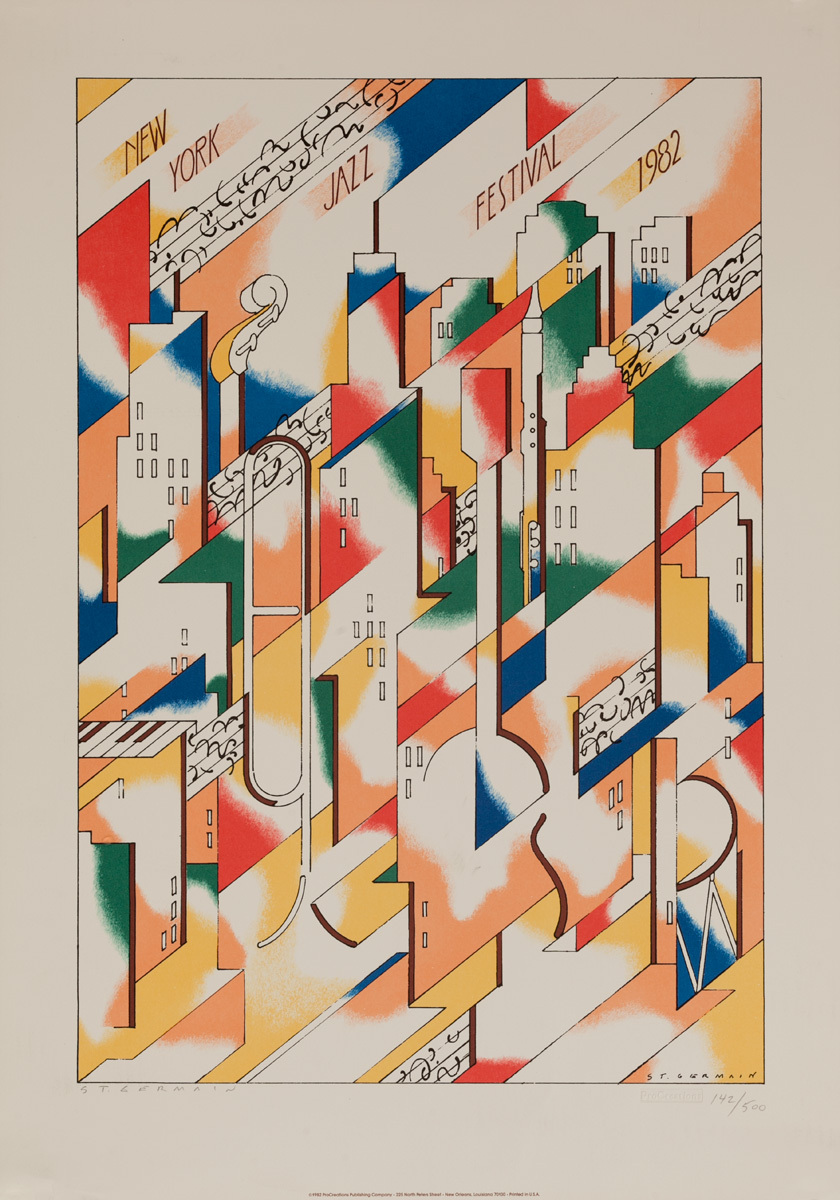The image is an abstract painting set against a white background, framed by a thin black border. The main rectangular space inside the border features a vibrant, multicolored depiction of a cityscape intertwined with musical elements. Skyscrapers, resembling New York landmarks, merge seamlessly with musical instruments such as trumpets and guitars, and streams of musical notes crisscross the scene. Bright colors of red, yellow, blue, green, orange, and white dominate the composition. Prominent text at the top reads "New York Jazz Festival, 1982." In the bottom right corner, the artist's signature appears alongside the edition number "142/500," suggesting it's part of a limited series.